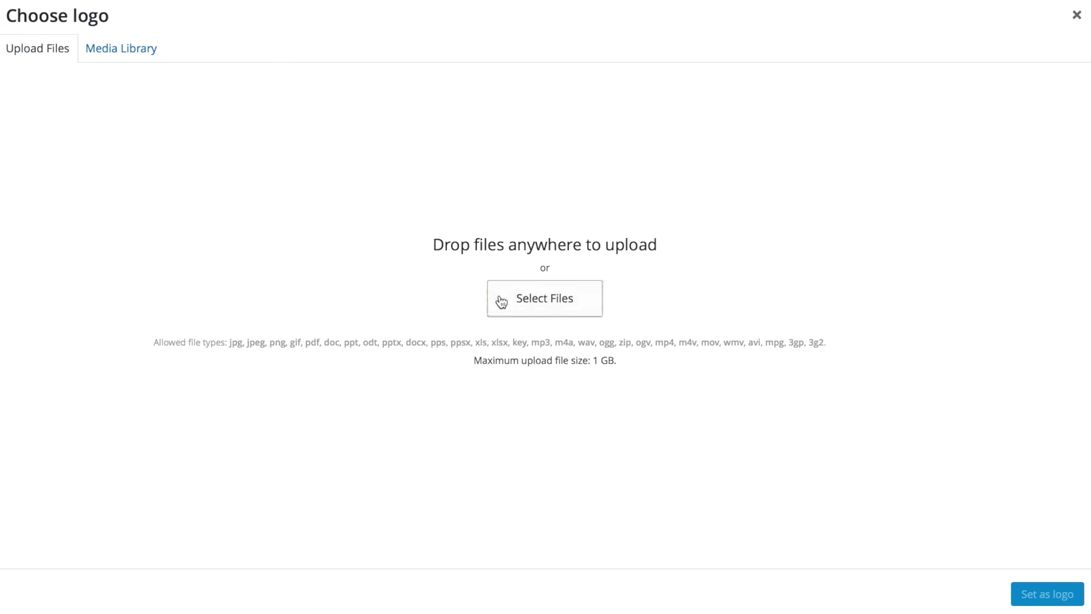This is a detailed screenshot from an unidentified software interface with a clean, white background. The top left corner displays several options, including "Choose Logo," "Upload Files," "Media Library," and "Drop Anywhere," along with instructions for uploading or selecting files. The allowed file types are listed and include various formats: JPEG, JPG, PNG, GIF, PDF, DOC, PPT, ODT, PPTX, DOCX, PPS, PPSX, XLS, XLSX, KEY, MP3, M4A, WAVE, OGG, ZIP, OGV, MP4, M4V, WMV, AVI, MPG, 3GP, and 3G2. It also specifies a maximum upload size of 1 GB. In the bottom right corner, there is a blue rectangular button labeled "Set as Logo." The image is purely textual and functional, with no photographic, animal, plant, vehicle, or aerial elements included.